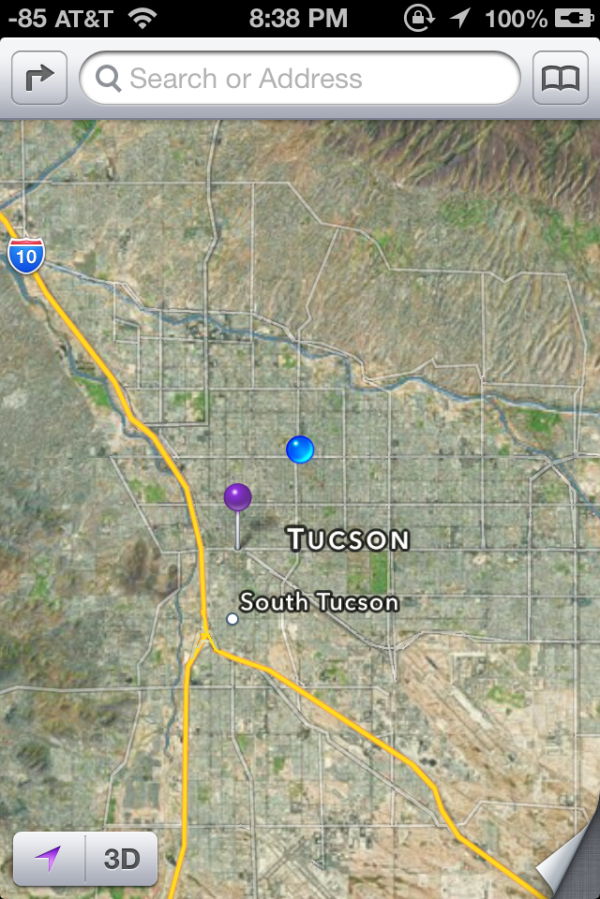This vertically rectangular image is a screenshot from a cell phone. At the very top of the frame, there is a horizontal black banner displaying the white text "AT&T", followed by the Wi-Fi signal icon. In the center of this banner, the current time "8:38 PM" is indicated, while additional icons and a fully charged battery icon (100%) are visible on the right side. Immediately below, a gray horizontal banner features a white search text field with the placeholder text "search or address."

The main portion of the image showcases a satellite view map. Interstate 10 is prominently displayed, running slightly vertically from the upper left, then angling slightly downward toward the center before forking into two separate directions. One fork continues downward to the left side of the frame, while the other angles toward the bottom right corner. A location, Tucson, is marked with a purple pin along this route. Beneath Tucson, the locality of South Tucson is pinpointed. In the bottom right corner of the map, a "3D" button is visible, likely allowing for a three-dimensional view of the map.